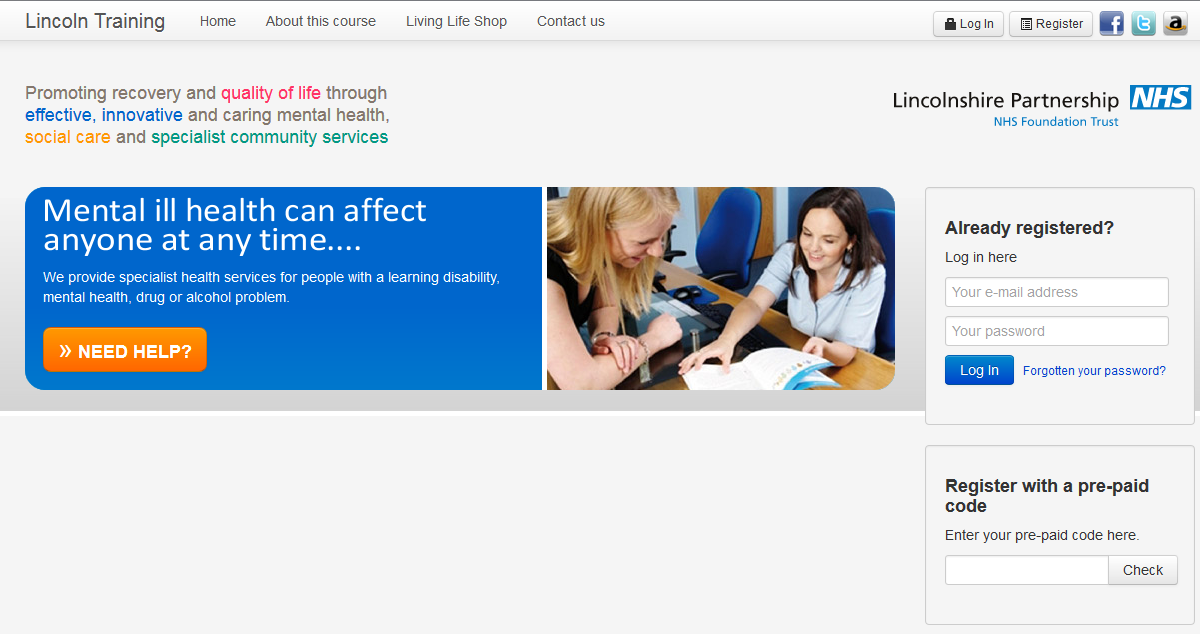**Screenshot Description: Lincoln Training Website**

The screenshot captures a section of the Lincoln Training website, showcasing its clean and straightforward design predominantly featuring a gray background. At the center, there's a prominent blue banner displaying a high-quality image of two women engaging collaboratively in what appears to be a business or educational setting.

**Details of the Website Layout**:
1. **Text and Colors**:
   - The website utilizes a mix of colored text in red, blue, yellow, and green alongside predominantly black text for general content.
2. **Header and Navigation**:
   - The top of the screen includes navigation options such as "Home," "About This Course," "Living Life Shop," "Contact Us," as well as "Log In" and "Register" buttons.
   - Additionally, icons for their Facebook, Twitter, and Amazon pages are available.
3. **Tagline**:
   - A prominent tagline at the top declares: "Promoting recovery and quality of life through effective, innovative, and caring mental health, social care, and specialist community services."
4. **Banner Details**:
   - Within the blue banner, there's a significant message stating: "Mental ill health can affect anyone at any time. We provide specialist health services for people with a learning disability, mental health, drug, or alcohol problem."
   - Following this informative message, there's an attention-grabbing orange button labeled "Need Help," inviting users to click for assistance.
5. **Login Area**:
   - There's an accessible area for users to log in to their accounts.

Overall, the detailed and thoughtful design of the Lincoln Training website underscore its commitment to providing essential mental health, social care, and specialized community services.